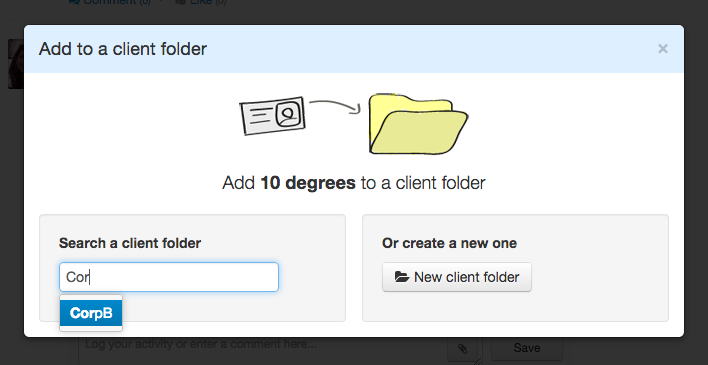In the center of the image, a dark background subtly supports the foreground content. On the bottom of this background, white text reads "Lock your activity or enter a comment here," adjacent to which is a blue "Save" button on the right.

Prominently displayed as a pop-up in the foreground, the header bar is blue with white text that reads "Add to a client folder." Below this header, the main content area features the instruction "Add '10 degrees' to a client folder." This section includes a yellow file icon along with a gray contact icon, which appears to be pointing towards the file icon, indicating the action of adding the contact to the folder.

Towards the lower portion of the pop-up, there are two distinct sections. On the left, the text "Search a client folder" appears above a search box containing the term "COR," with the cursor placed at the end. Directly beneath the search box is a blue-highlighted suggestion "CORPB."

On the right side, the text "Or create a new one" is displayed above a gray button labeled "New client folder" in black text. The overall layout is organized and directs the user clearly through the process of adding a contact to a client folder or creating a new one.